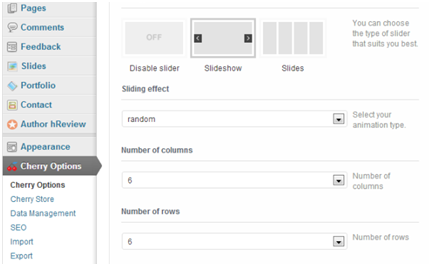This color image features a detailed screenshot of a website interface predominantly set against a white background with text in gray, black, and blue fonts. The screenshot is wider than it is tall, suggesting it was likely taken on a computer rather than a phone.

On the left side of the screenshot, a vertical menu lists various options or commands. The menu items include "Pages," "Comments," "Feedback," "Slides," "Portfolio," "Contact," "Author," "HReview," "Appearance," and the currently selected option, "Cherry Options," which is highlighted in dark gray with red accents. Under "Cherry Options," other selectable items include "Cherry Store," "Data Management," "SEO," "Import," and "Export."

In the center and right portions of the screenshot, the top-right section includes a prompt stating, "You can choose the type of slider that suits you best." Below this prompt are three graphical choices for the slider settings, each with descriptive text:

1. **Disable Slider**: Represented by a gray rectangle labeled "Off."
2. **Slide Show**: Indicated by a gray rectangle with arrows on either side.
3. **Slides**: Depicted as a series of four gray vertical rectangles.

Further down, there is a menu for selecting sliding effects, with "Random" being the chosen animation type. Beneath this menu, settings for the layout are visible:
- The number of columns is set to six.
- The number of rows is also set to six.

This detailed interface allows the user to customize various aspects of their website, from slider types and animations to the structural layout of their content.